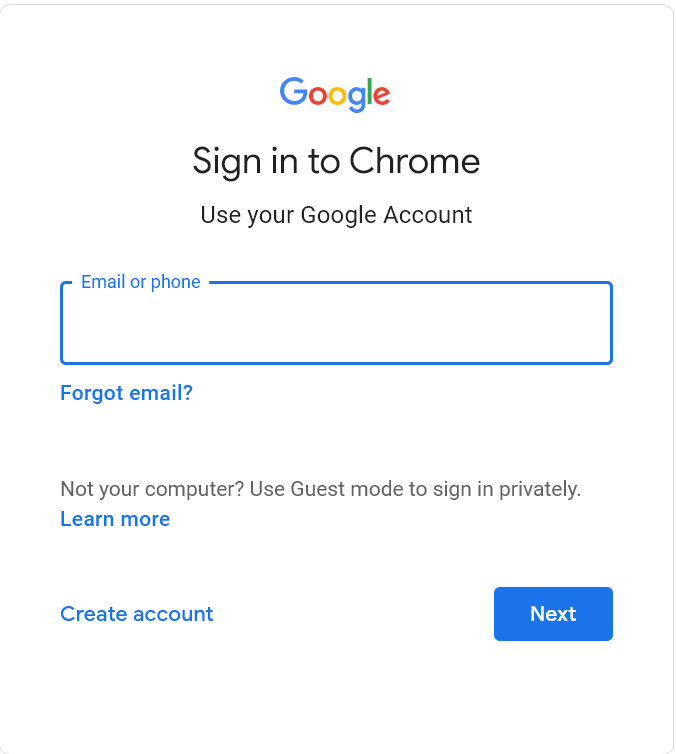A screenshot of a Google login screen is shown. The interface is framed by a thin, dark grey border. Centered at the top is the Google logo, composed of a multi-colored 'G' in blue, a red 'O', an orange 'O', a lowercase blue 'g', a green 'l', and a red 'e'. Below the logo, in bold black text, it reads "Sign in to Chrome," followed by smaller bold text stating, "Use your Google Account."

Further down, there is a prominently positioned, dark blue rectangle with an open top-left corner. Inside the rectangle, placeholder text reads "Email or phone." Just below this field and outside the rectangle, there is a "Forgot email?" link in bold blue text.

Beneath this section, there is a brief white space followed by a black text prompt: "Not your computer? Use Guest mode to sign in privately." To the right of this message, there is a "Learn more" hyperlink in bold blue text, and next to it, another hyperlink that says "Create account."

Positioned below these hyperlinks, slightly to the right, is a dark blue rectangular button with the white text "Next." The left edge of the image appears to be slightly truncated.